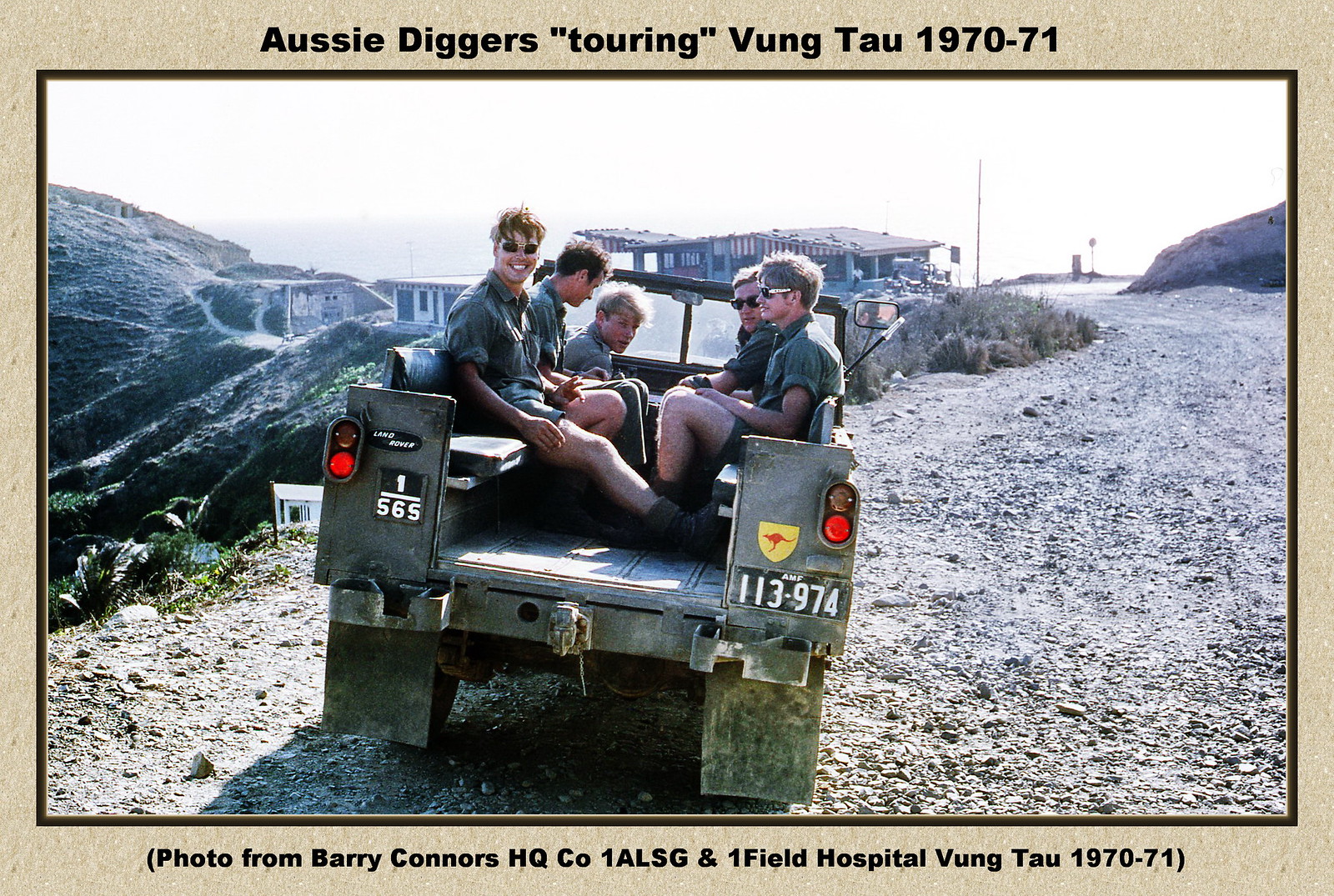The image is a vintage photograph from the Vietnam War era, specifically from 1970-71, depicting an outdoor scene with five young men sitting in the back of a military jeep. The photo features a tan border with black text at the top and bottom. The top border states: "Aussie diggers (touring) Vung Tau 1970-71," while the bottom border credits the photo to "Barry Connors HQ CO 1ALSG and One Field Hospital, Vung Tau 1970-71."

In the center of the image, the jeep is facing slightly to the right, with its rear end visible. There's a bench on each side in the back of the jeep, with three men seated on the left and two on the right. The man closest to the viewer on the left has curly brown hair, glasses, and is smiling. Across from him, on the right side, is another man wearing glasses and looking back at the first man. All the men are dressed in matching green tops and shorts, typical soldier uniforms, with their bare legs visible.

To the left of the jeep, there is an edge of a steep hill that slopes downward, while on the right, a rugged gravel road curves up and then around. In the backdrop, a small building is partially visible amidst some shrubs and wispy grass, adding to the rustic and rugged atmosphere of the scene. Small hills can be seen in the distance, contributing to the dry and bright valley setting, making the environment appear somewhat harsh and austere.